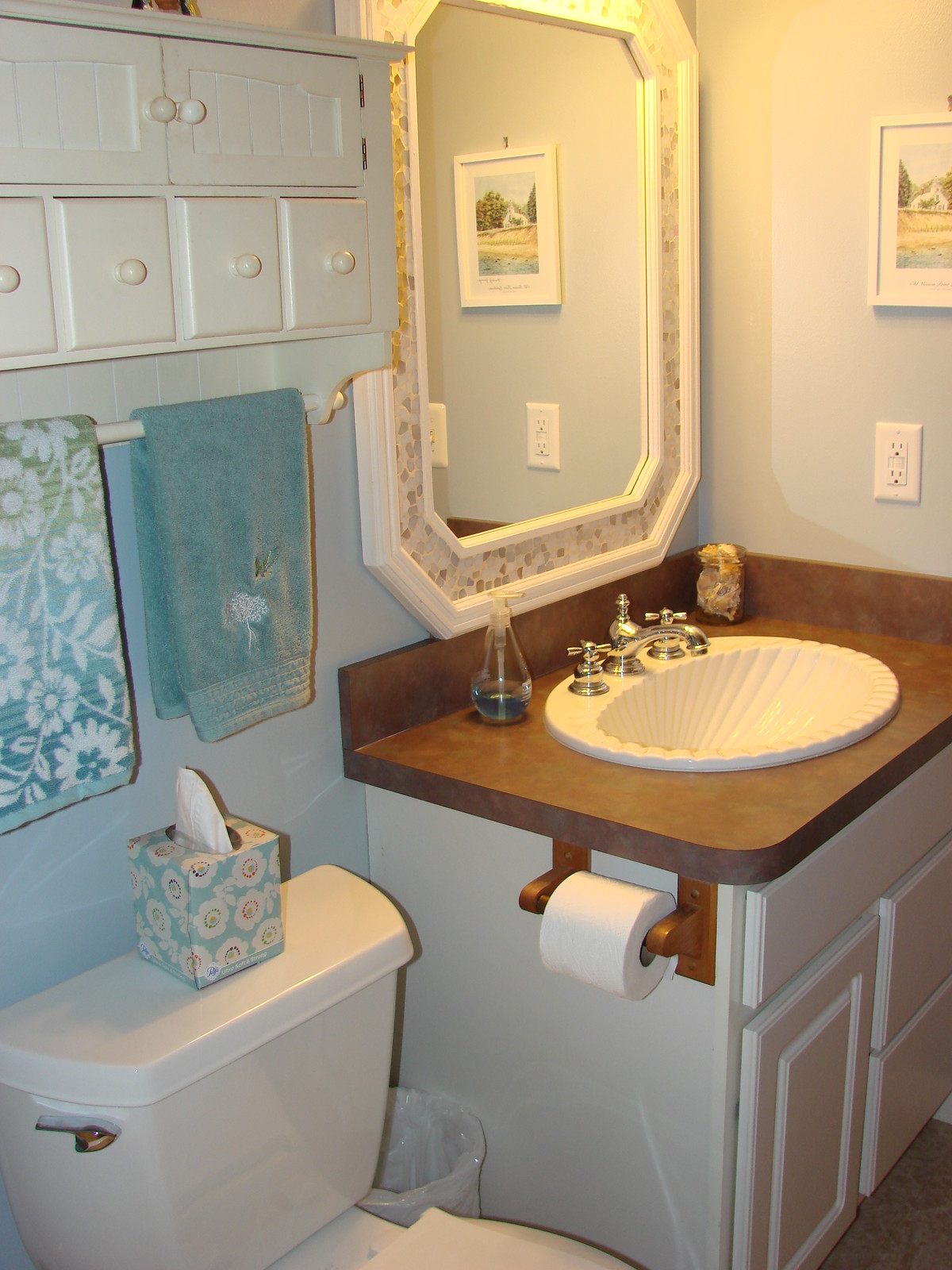The bathroom depicted in the image exudes a slightly dated aesthetic, characterized by its dark brown laminate countertop. The sink is notably shell-shaped, featuring intricate lines and puff-like details that mimic the appearance of a real shell. Contemporary fixtures, which appear relatively new, contrast with the overall vintage feel.

Prominently displayed above the sink is a large mirror embellished with a tan mosaic border, adding a touch of elegance to the space. A nearly empty bottle of soft soap is placed on the counter. Adjacent to the mirror, there's a small picture frame showcasing an image of a house, a tree, and a body of water, contributing a quaint charm to the room.

In the toilet area, a set of white cabinetry is mounted above the toilet, consisting of drawers and two large doors. The drawers are equipped with small knobs, while the lower part of the cabinetry integrates a towel rack. Hanging from the towel rack are two turquoise towels: one featuring a simple design, and the other adorned with floral and leaf patterns. A white tissue box is stationed on the toilet's cistern, which complements the white cabinets and toilet. Mounted on the side of the cabinet is a wooden toilet paper holder. Completing the scene is a garbage pail lined with a plastic bag.